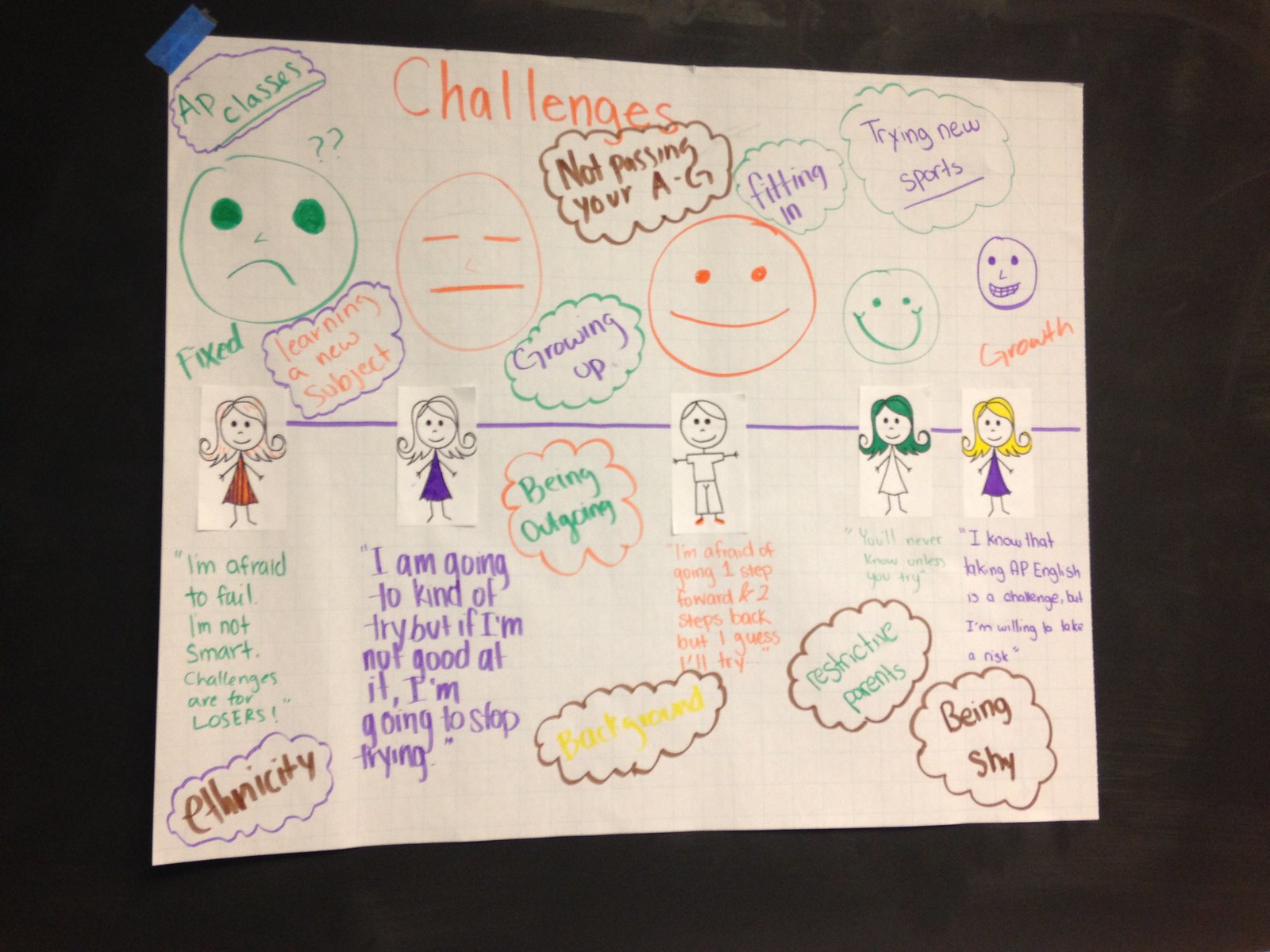This photograph showcases a detailed school project, visually representing a student's anticipated challenges and corresponding emotions through an illustrated emotional timeline. At the top of the drawing, the word "Challenges" is prominently displayed in red colored pencil or crayon. Below this title, an array of expressive circle faces spans horizontally from left to right, transitioning from a sad face at the leftmost edge to an extremely happy one on the far right.

The first face, depicted with a downward-curved mouth, conveys sadness. The next face features horizontal lines for eyes and a neutral straight line for a mouth, showing indifference. Progressing rightwards, the subsequent face in red has slightly upward-curving eyes and mouth, depicting mild happiness. Further right, a green face illustrates a deep smile, while the final purple face exhibits a wide, toothy grin representing extreme happiness.

Beneath this row of emotive circles, the project further elaborates with cartoon illustrations of four women and a boy, interconnected by a dark line, suggesting the boy is central to these interactions. Written text in marker or colored pencil appears below each cartoon figure, though most of it is difficult to decipher. Below this text, several clouds are tilted left, each containing more written reflections.

In the student’s visualization, each emotional state is accompanied by thought-provoking quotations capturing their mindset as they face various life challenges. The timeline starts with a quote in the sad section saying, “I am afraid to fail. I'm not smart. Challenges are for losers." It transitions towards a more neutral sentiment, “I am outgoing. I am going to kind of try but if I'm not good at it I'm going to stop trying." Moving into the happier stages, the quotes express growing optimism, “I’m afraid of going one step forward and two steps back but I guess I will try,” followed by, “You never know until you try.” The happiest emotion culminates with, “I know that taking AP English is a challenge but I'm willing to take a risk.”

Together, these elements provide a comprehensive narrative of the student's journey, depicting their apprehensions, growth, and positive outlook, especially focusing on the challenge of taking AP English and their desire to succeed.